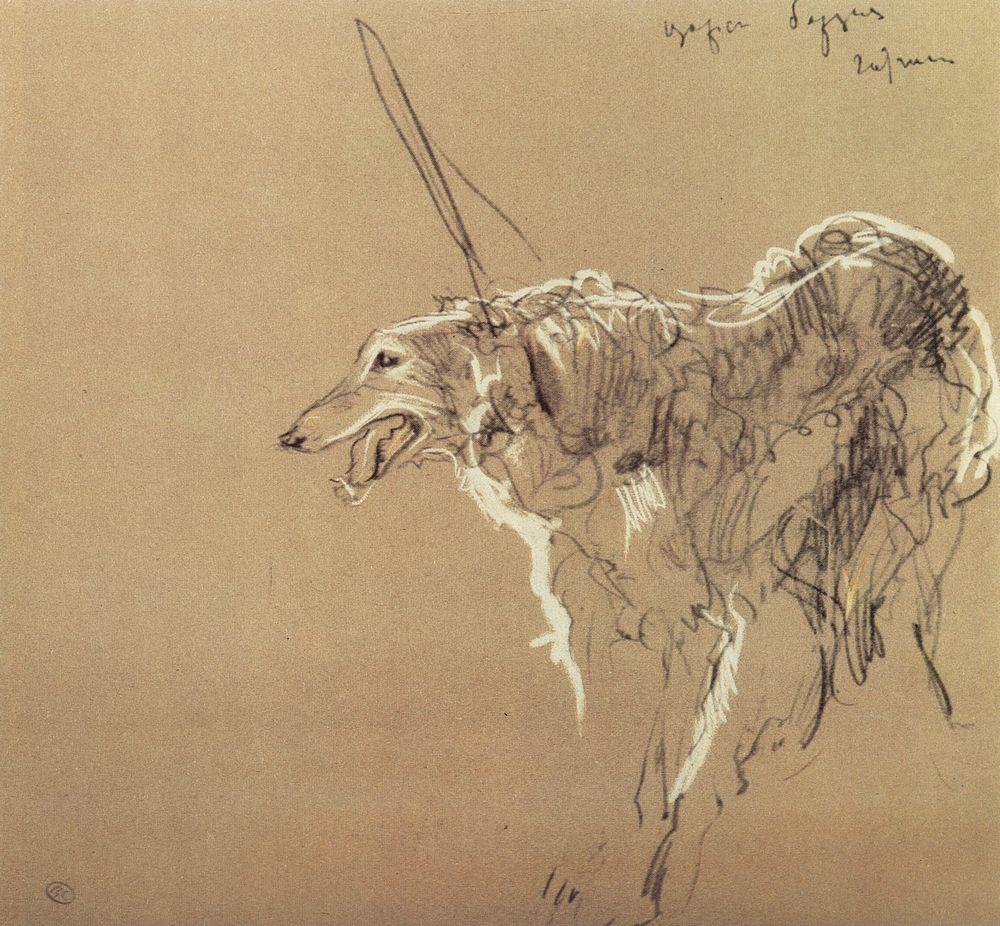This is a detailed black ink and pencil sketch on a tan, peach-colored background, depicting a dog that appears to be a greyhound or a long-haired greyhound. The dog is facing left, its mouth open with its tongue partially hanging out, showcasing its teeth. The sketch varies in detail, with the head being the most defined part of the drawing, while the body, legs, and tail are rougher and more suggestive, giving the impression that the sketch is incomplete. A leash is also sketched in. There is some cursive writing at the top right of the image, possibly a signature or name, although it’s difficult to decipher. Additionally, there is a circle with what might be initials in the bottom left corner of the image. The only colors used in the sketch are black and white, adding to its minimalistic and somewhat abstract quality.